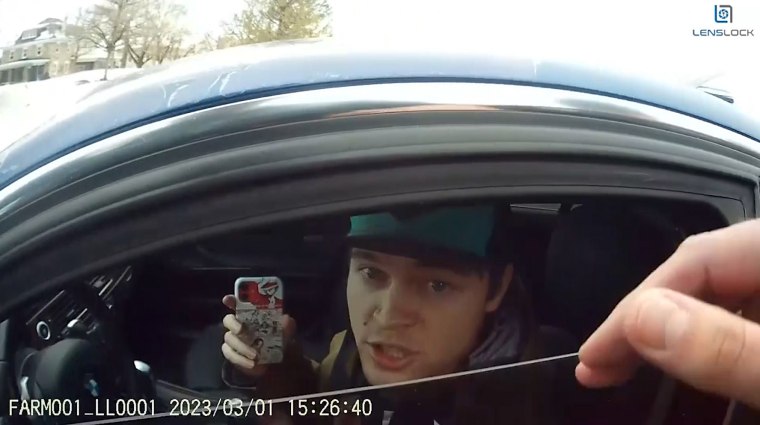This image, likely a screen grab from a body camera, captures a daytime scene during winter, as indicated by snow-covered surroundings and bare trees in the background. It features a young Caucasian man, seated in the driver's seat of a light blue car, wearing a black and green baseball cap. He holds an iPhone with a white case, possibly featuring cartoon characters, in his right hand. The man has his mouth open, appearing to speak to someone outside the vehicle. In the bottom right corner of the image, the hand of a person, presumably a police officer, is visible, with their thumb and two fingers extended. The lower left corner of the image displays camera notations: "FAR M001_LL0001 2023-03-01 15:26:40." An upper right watermark shows a partially closed green box with the text "LENSLOCK" in capital letters beneath it. Colors in the image include blue, green, white, red, black, and silver.